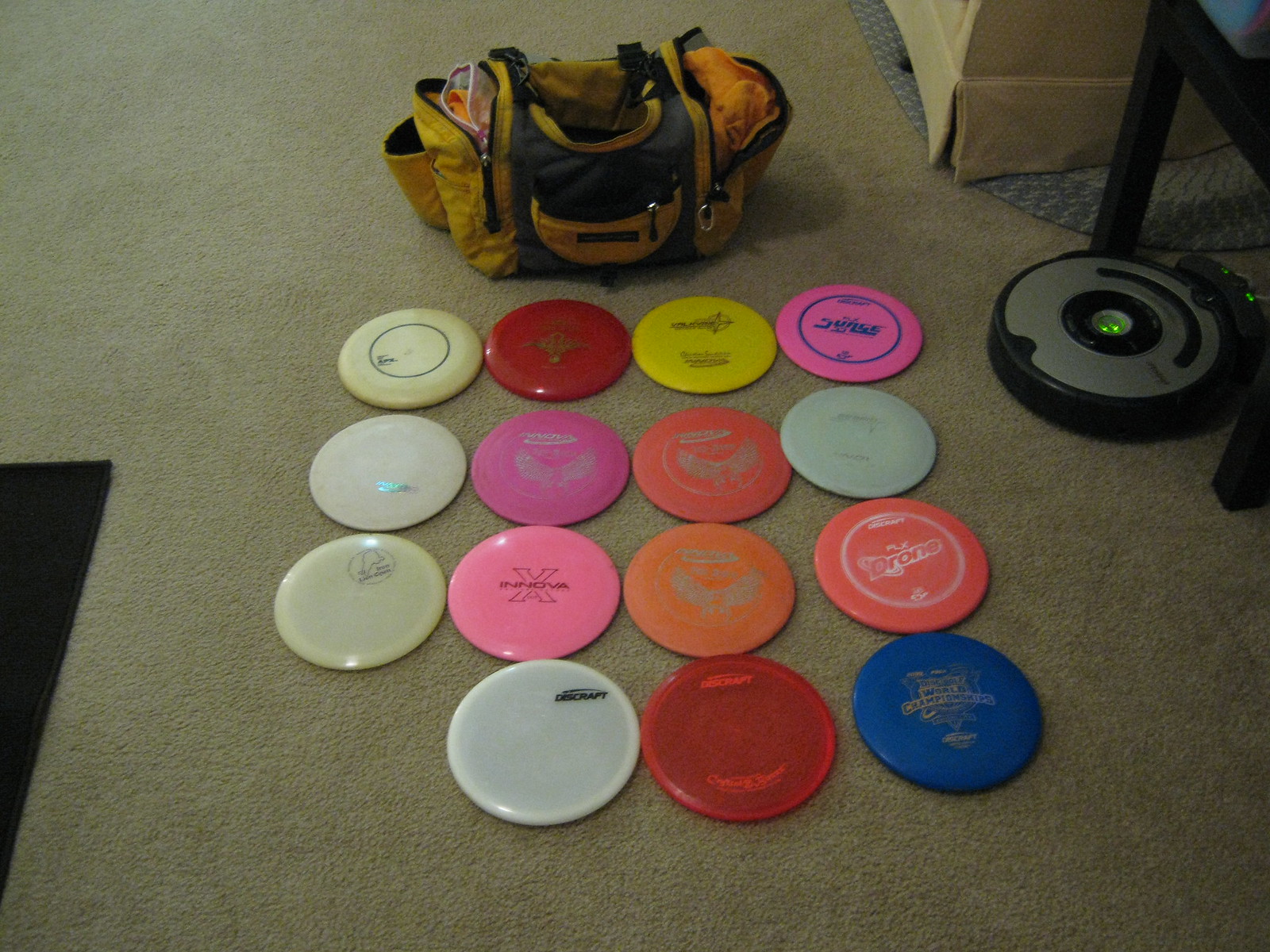This indoor photograph captures a neatly arranged assortment of 15 Frisbee golf discs of various vibrant colors placed on a light beige carpet. The discs are organized into four rows: the top row includes a white, red, yellow, and pink frisbee; the second row features a white, pink, orange, and light blue frisbee; the third row consists of white, pink, and two orange frisbees; and the bottom row has a white, red, and blue frisbee. Each disc displays some form of ornate design or branding text, mostly in black or white, though the details are not clearly readable.

In the upper middle of the image, a brown duffel bag with unzipped sides revealing some internal bags is present, hinting at its use for carrying these frisbees for Frisbee golf. To the right of the discs is a robot vacuum designed for carpet cleaning, characterized by a black edge and a gray top. Additionally, the upper right corner of the photo reveals part of a cream-colored piece of furniture alongside a dark black wooden table. The scene is softly lit, accentuating the indoor, homey setting.